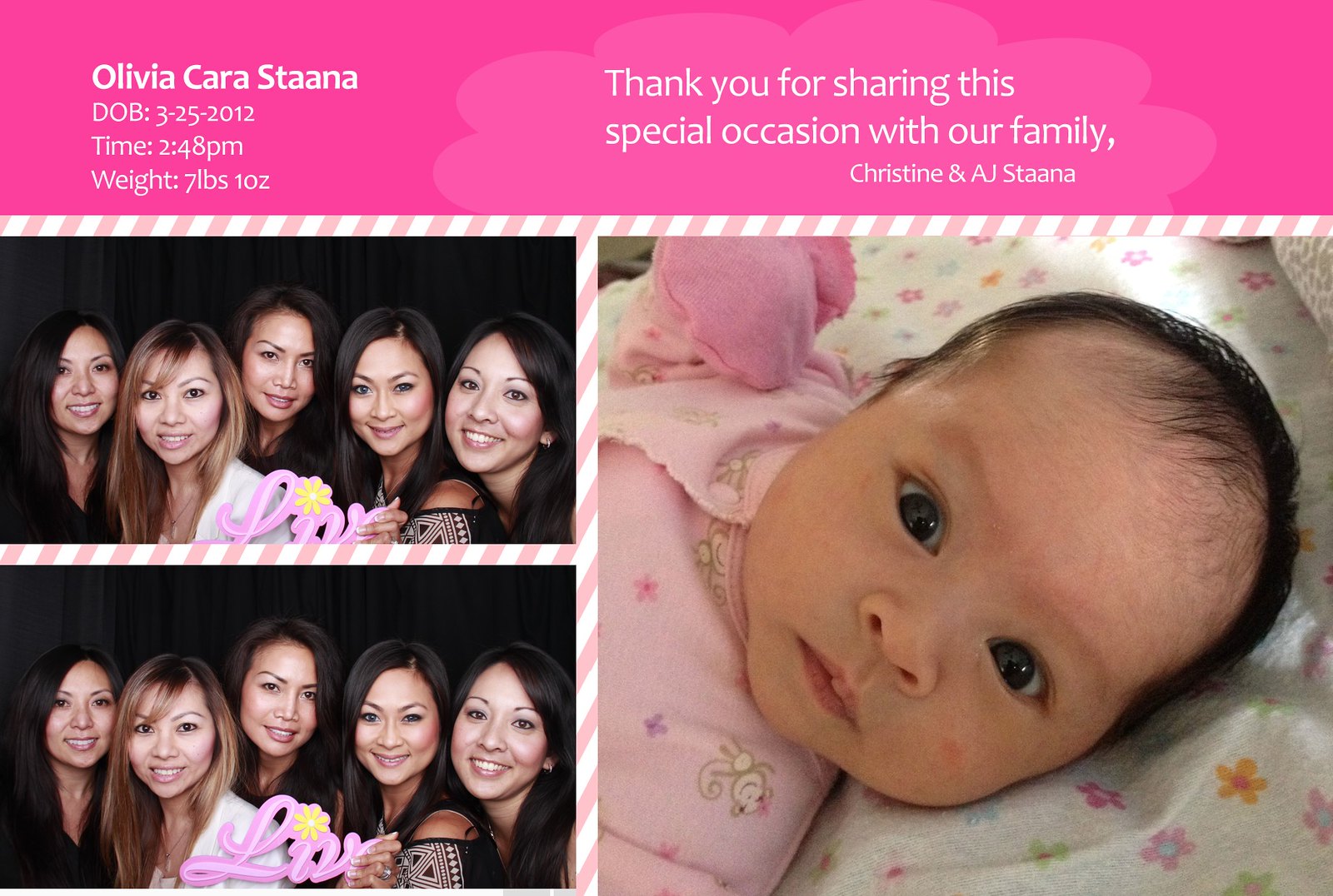This vibrant birth announcement features a bright pink background adorned with white text. A pink banner stretches across the top, prominently displaying the name "Olivia Kara Stana," the date of birth "3-25-2012," the time "2:48 PM," and the weight "7 pounds, 10 ounces." Below this information is a heartfelt message: "Thank you for sharing this special occasion with our family, Christine and AJ Stana."

On the right side of the announcement, a larger picture showcases baby Olivia, dressed in a pink onesie with pink and purple flowers and little brown monkeys, lying on her side on a white blanket decorated with orange, pink, and green flowers. To the left, two smaller images depict a group of five women with four having dark hair and one with lighter hair. These women appear twice, once positioned below the other, dressed predominantly in black clothing, with one woman in white adorned with a pink and yellow flower accessory. Separating the images are slanted white and pink stripes, adding a whimsical touch to the announcement.